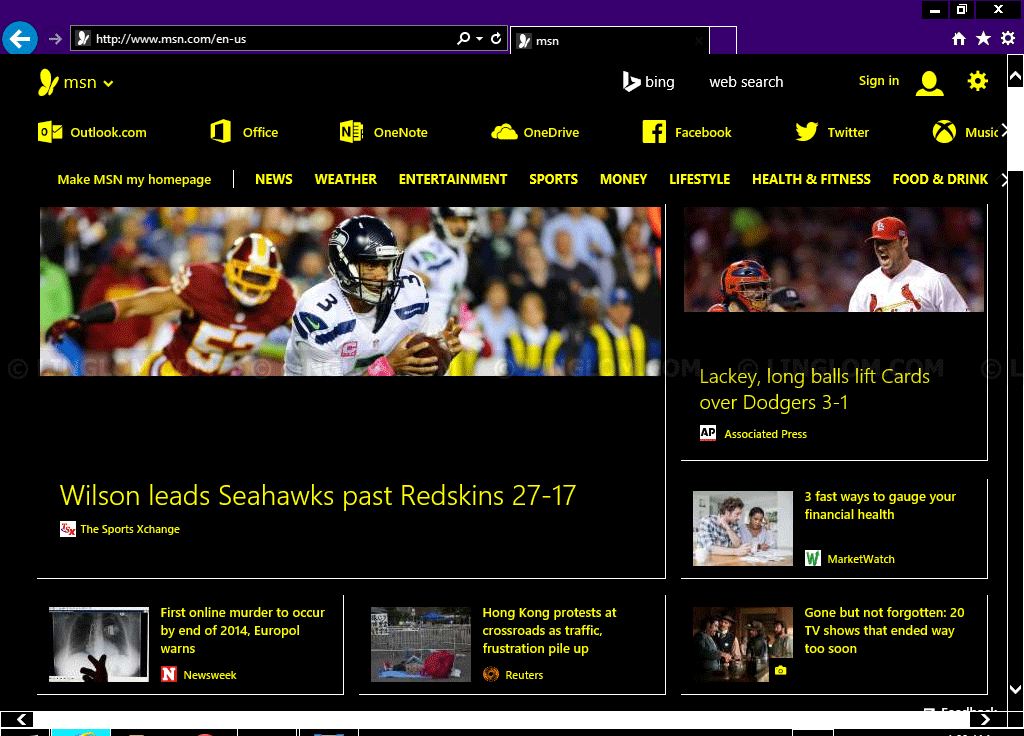The image showcases the MSN.com homepage. At the top, the address bar, rendered in black, reads "MSN.com/EN-US." To its left is a blue back arrow icon and a gray forward arrow icon. A tab labeled "MSN" is open, and on the right side of the address bar are three white icons: a house, a star, and a gear, signifying Home, Favorites, and Settings respectively. Beside these are the window control buttons—minimize, maximize, and close.

Below the address bar, the page prominently displays the MSN logo in yellow. Directly beneath it are links to several services: Outlook.com, Office, OneNote, OneDrive, Facebook, Twitter, and Music. Another link encourages users to "Make MSN My Homepage." The navigation bar lists various categories: News, Weather, Entertainment, Sports, Money, Lifestyle, Health & Fitness, and Food & Drink.

The main content area is filled with images and headlines. The largest feature highlights a football game, with an image of a player carrying a football while another player chases him. The caption reads, "Wilson leads Seahawks past Redskins 27-17," attributing the news to Sports Exchange.

Adjacent to this, another section reports, "Lackey long balls lift Cards over Dodgers 3-1," illustrated with a photograph of a baseball game in action. Below these major articles, additional headlines are listed:
- "Three fast ways to gauge your financial health"
- "First online murder to occur by end of 2014, Europol warns"
- "Hong Kong protests at crossroads as traffic frustration piles up"
- "Gone but not forgotten: 20 TV shows that ended way too soon"

Each headline is accompanied by a corresponding image, making the page visually engaging and information-rich.